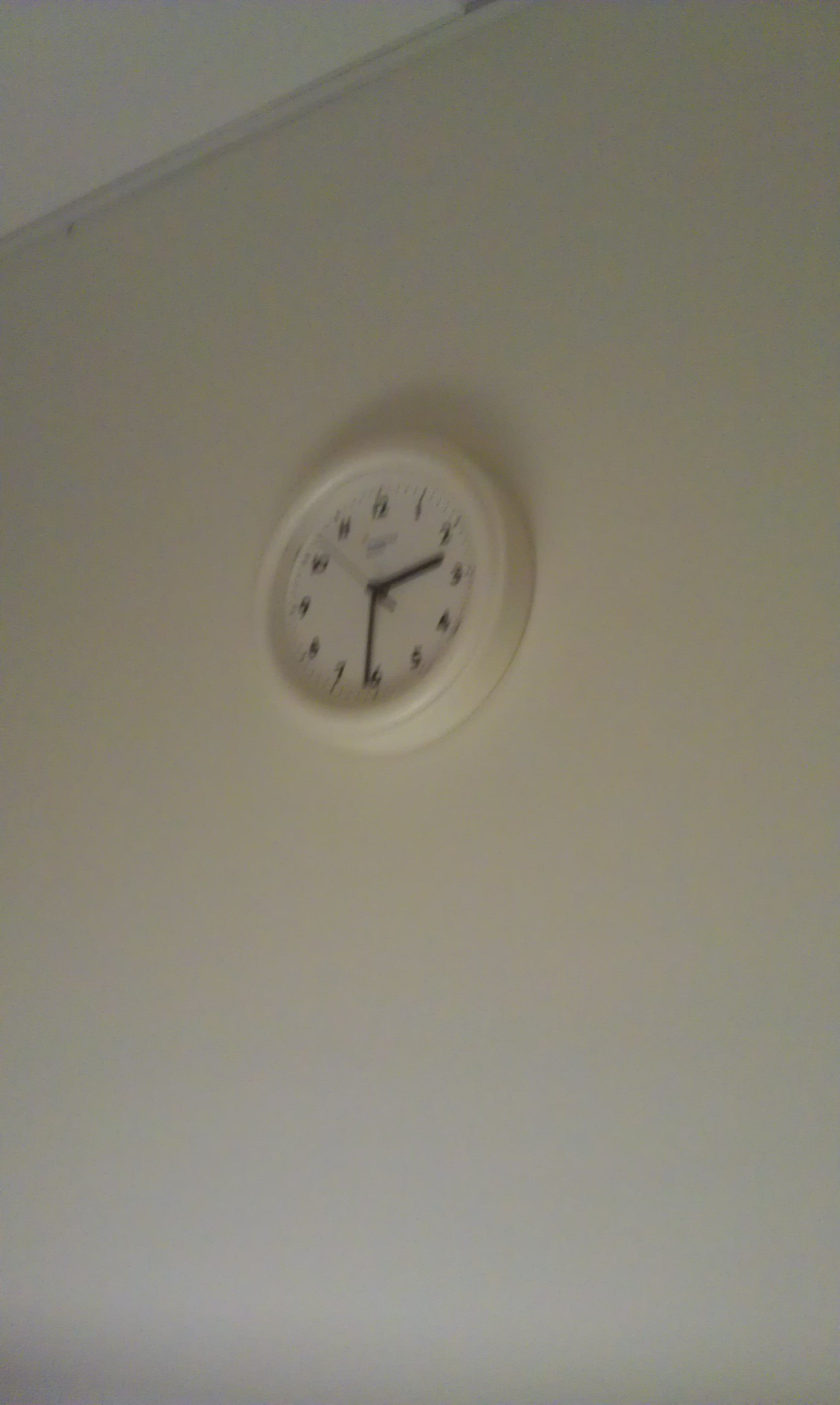The image depicts a minimalist scene where a white manual clock is affixed to a blank wall that meets the ceiling at the top left corner of the frame. The wall and the ceiling are both very light in color, almost white, though the wall appears slightly darker due to shadows and low lighting. The clock itself has a white frame with a black face, black hands, and black numbers marking the traditional 1-12 hours. The larger hand points to the 6, the smaller hand between the 2 and 3, and the second hand near the 10, indicating the time is approximately 2:31pm. The photograph, likely taken with a phone camera given its mediocre quality and slight blurriness, evokes a rather dull and uninspired atmosphere due to the lack of lighting and clear detail. The overall composition suggests a clean yet unremarkable space, perhaps reminiscent of a classroom or a similarly sterile environment.